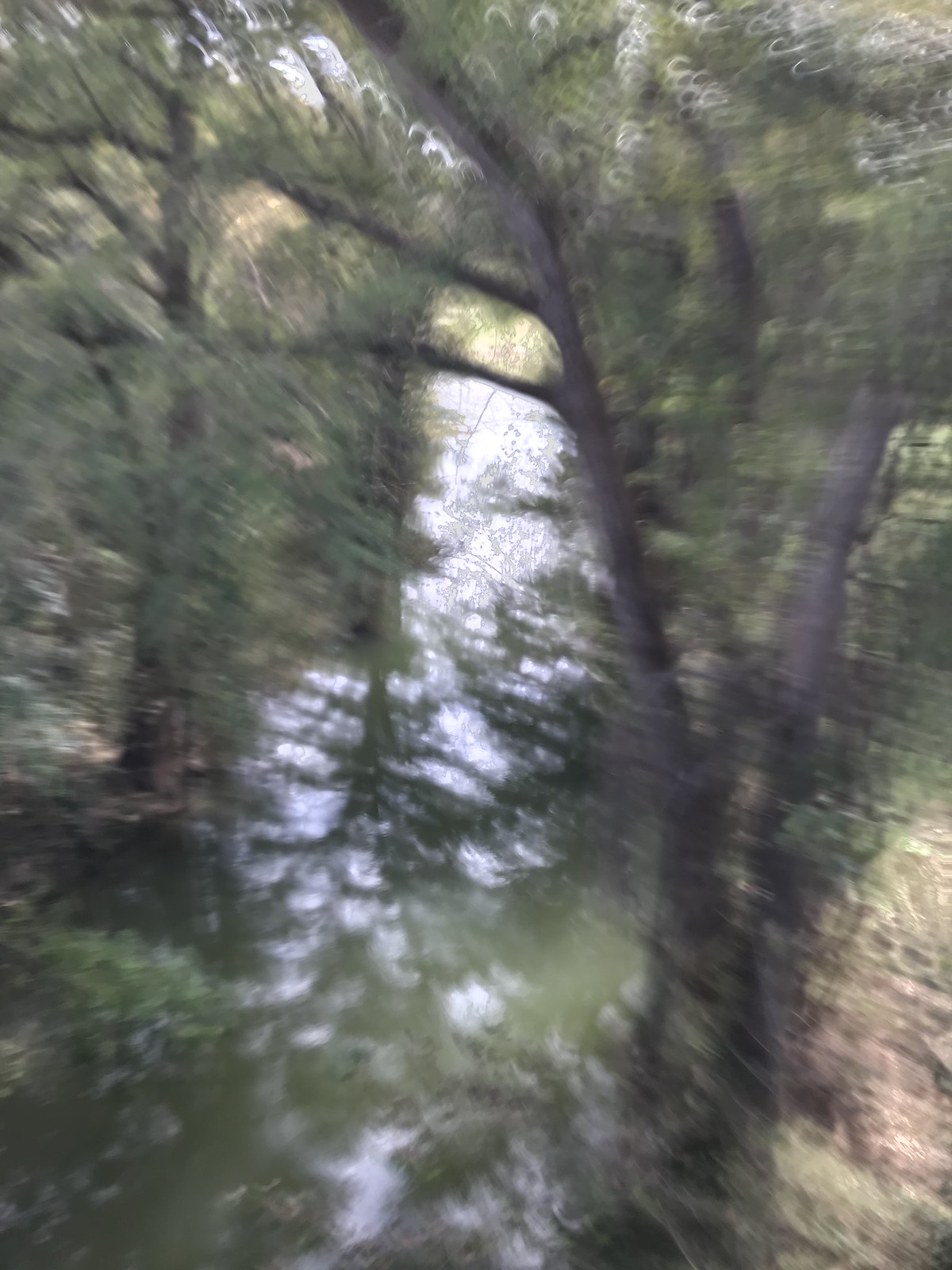The photograph depicts a blurry scene of a forest with predominantly dark evergreen tree trunks and branches in the foreground. Through the foliage, there appears to be a river running through the middle of the forest, catching reflections of the surrounding trees and sky. The image has a doubling or ghosting effect, creating the illusion of motion and making details difficult to discern. Despite the blurriness, some bright spots of sky peek through the tree canopy, indicating it is daylight, likely overcast as the light permeates the greenish-brown river water. Bushes and various types of foliage scatter throughout the dense forest scene, adding to the rich natural texture of the photo.